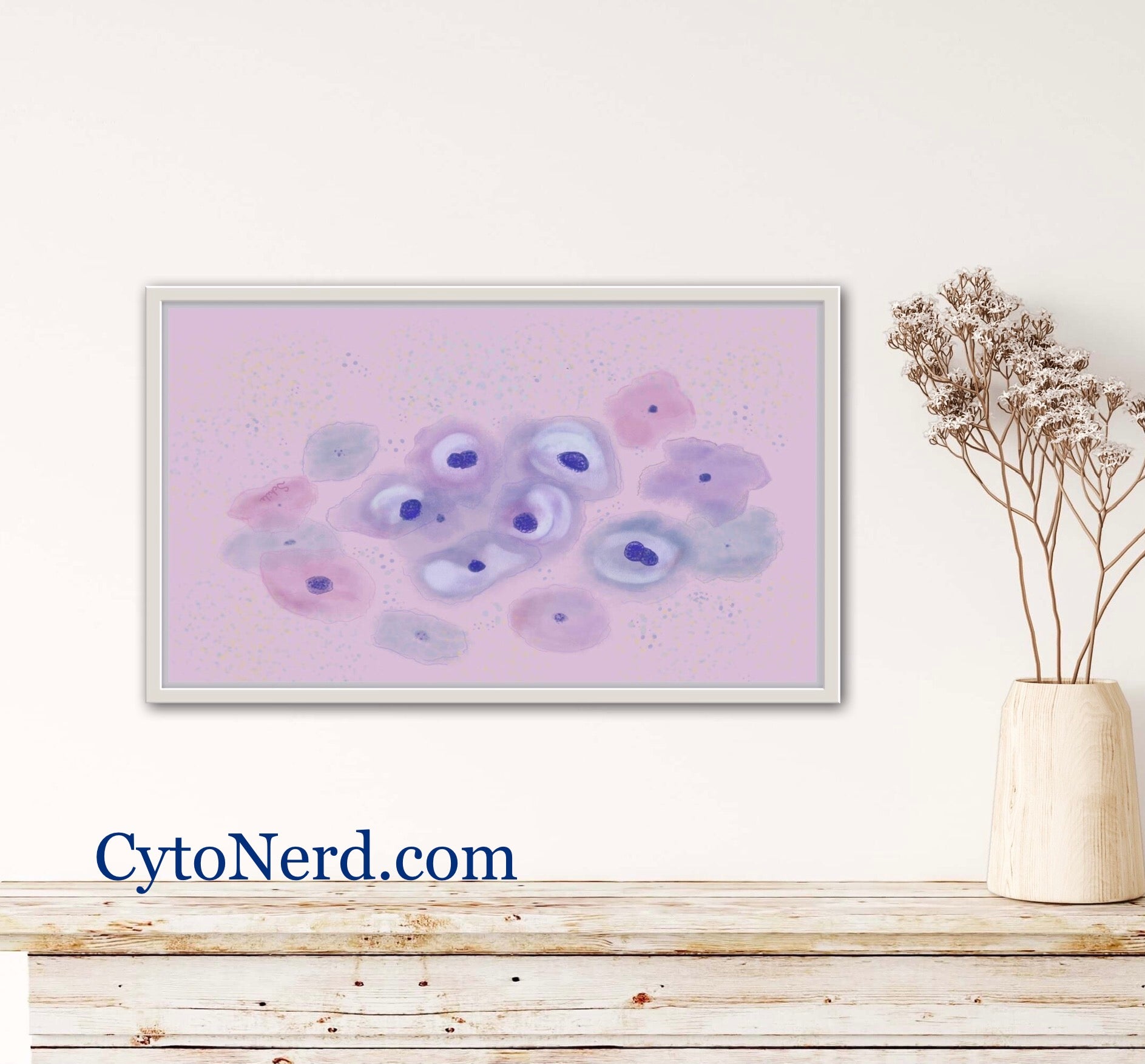The image is a stylish advertisement for the website Cytonerd.com, featuring a cozy interior scene dominated by a beige wall as the backdrop. A piece of art hangs centrally on this wall, framed by a subtle silver or celadon light green border. The artwork itself showcases an abstract representation of cytoplasm with a light pink background adorned with various blotches of purple and darker pink hues.

Beneath the art piece is a substantial wooden mantel, rustic in appearance and crafted from natural wood. To the right of this mantel, there is a blonde oak vase prominently featured, containing dried, slender brown foliage that adds a natural touch to the decor.

Hanging adjacent to or directly on the mantle are the boldly displayed words "Cytonerd.com" in blue ink, clearly marking the website being advertised. The entire composition is carefully balanced, with harmonious earthy tones and a scientific theme subtly intertwined through the design elements.